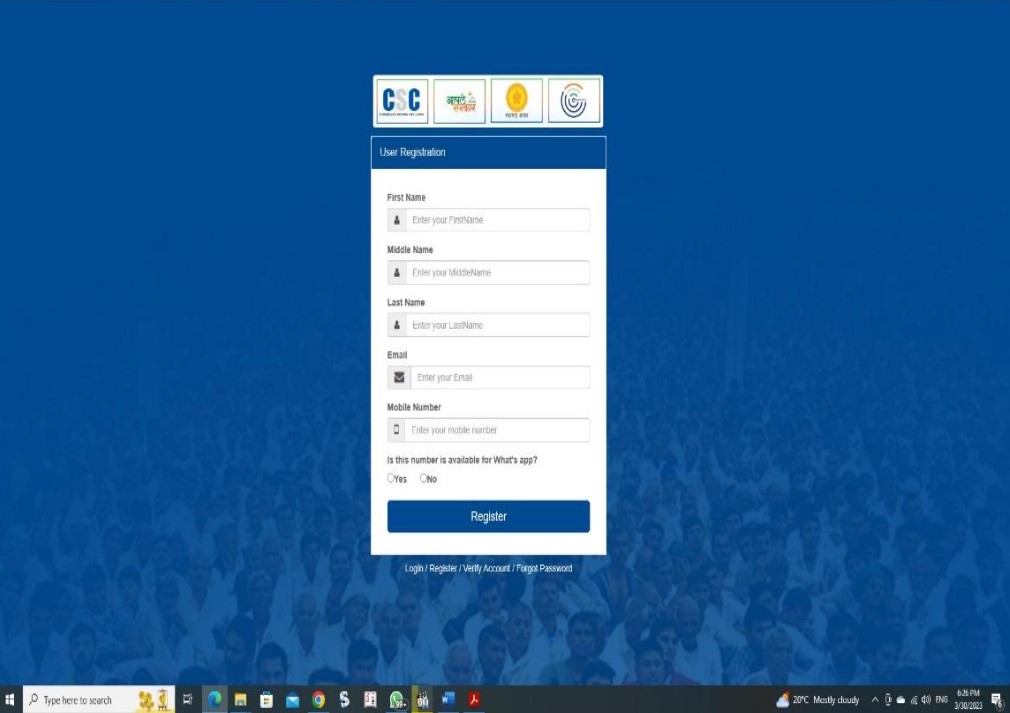The image features a user registration form set against a dark blue background that subtly fades into a large crowd at the bottom, all dressed in white. Dominating the center of the image, a rectangular form has a dark blue header labeled "User Registration" in white, positioned toward the left. 

The form includes several fields for user input, each bordered by a light gray outline. The first field is for "First Name" with a gray italic placeholder text reading "Enter your first name." To the left of the input box, a small gray square contains a user icon. A similar format is followed for the "Middle Name" and "Last Name" fields.

Following these, an "Email" field is presented, distinguished by an envelope icon in the square area to the left. Next, the "Mobile Number" field appears, marked by a mobile phone icon. Beneath this, a statement in black text asks, "Is this the number available for WhatsApp?" with two circular checkboxes labeled "Yes" and "No," both unselected.

At the bottom of the form, a long, dark blue button matching the background displays the word "Register" in white. 

At the very bottom of the image, a taskbar is visible. On the far left is the slanted Windows logo, giving a 3D effect of moving forward. Next to it is a search bar that reads "Type here to search." To the right, a gold leafy object and what appears to be a bird cage are visible. To the far right are several icons, including Microsoft Edge (which is currently selected), a folder, the Microsoft Store logo, and an envelope indicating email access.